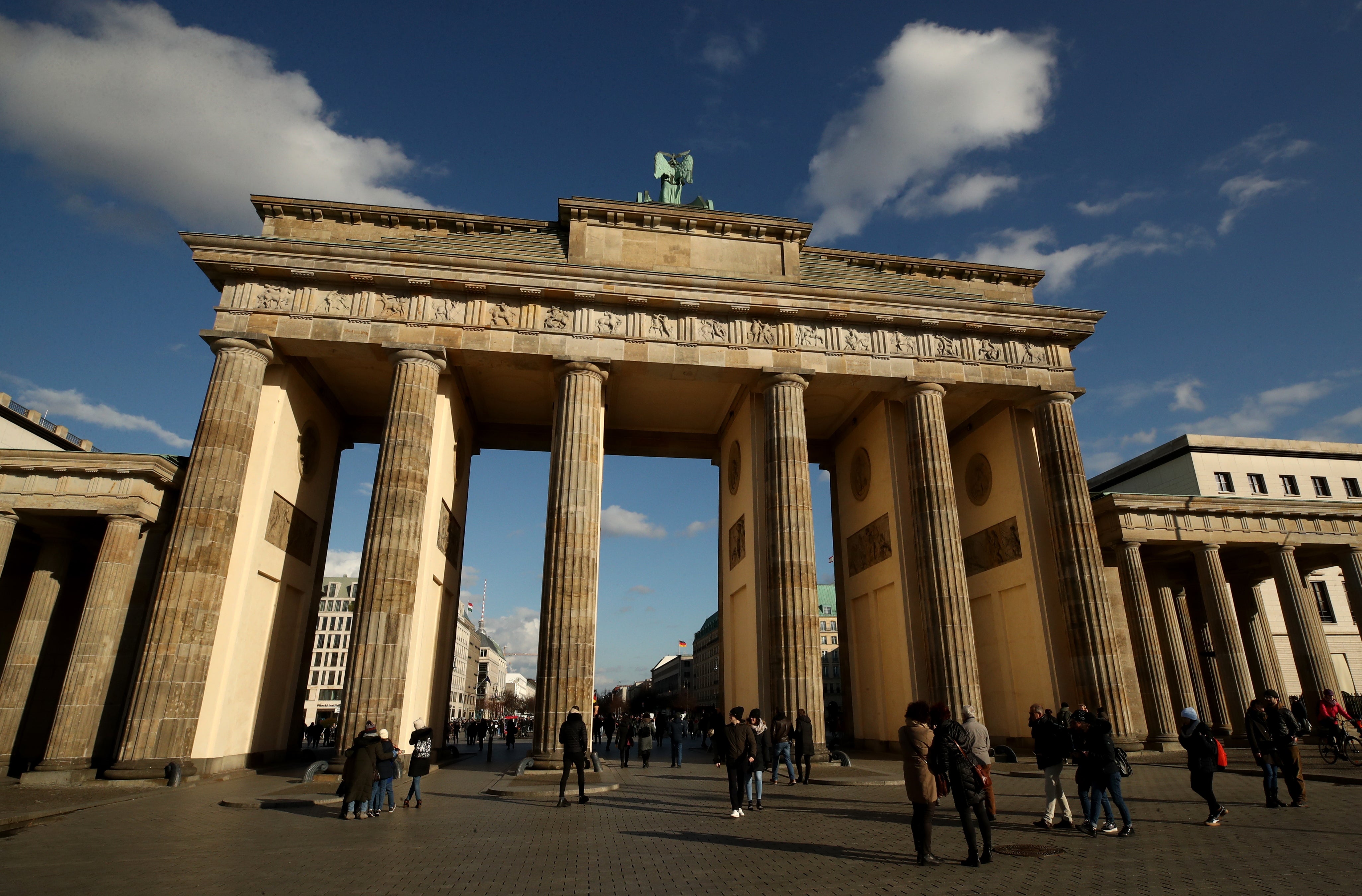The image captures a bustling city square, possibly a well-known tourist spot in Germany, given the visibility of a German flag in the distance. Dominating the scene is an imposing ancient archway, supported by six tall columns and capped by detailed stonework featuring various images. Atop this archway stands a weathered green statue of an angel, suggesting it may have once been a different color before the elements altered it. Flanking the archway are two smaller, yet similar, structures, each mirroring the design of the main arch but on a smaller scale. The ground is paved with grey stones, crowded with people who are either admiring the architectural grandeur, walking through the archway, or simply strolling the vicinity. Around the square, numerous stone buildings add to the historic ambiance, all under a clear blue sky dotted with white clouds.